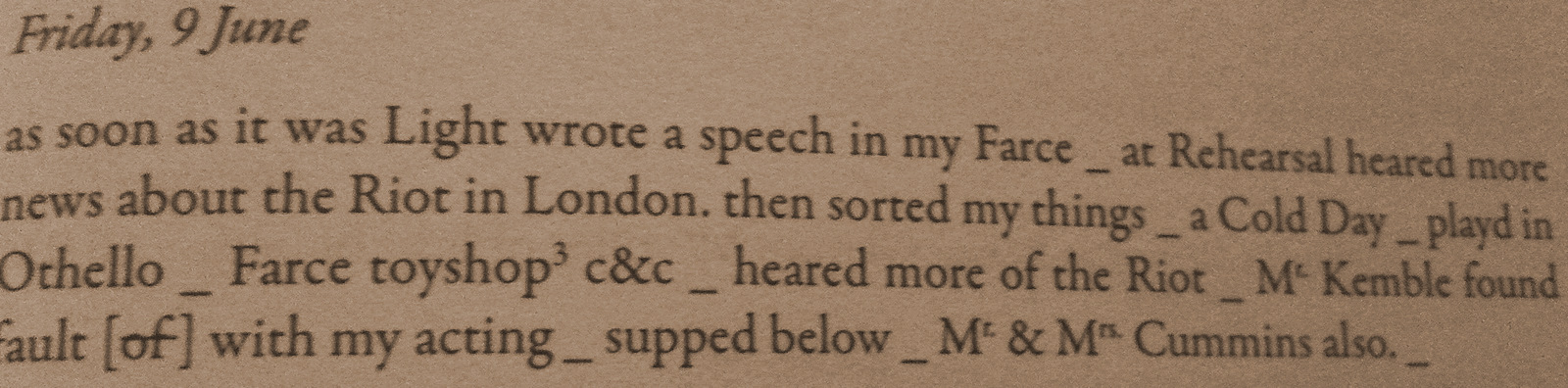The horizontally oriented photograph captures an excerpt from a diary printed on a light brown page with darker brown text. In the top left corner, the text reads "Friday, 9 June." Beneath this heading, the entry begins: 

"As soon as it was light, wrote a speech in my farce, then at rehearsal heard more news about the riot in London. Sorted my things. A cold day, played in Othello. Farce toy shop, C&C. Heard more of the riot. McKimble found fault with my acting. Supped below. Mr. and Mrs. Cummins also."

Key elements are denoted by underscores, suggesting emphasis or breaks in the text.